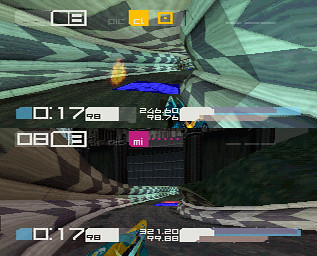A screenshot taken from an old-school racing video game in split-screen mode. The screen is divided into two sections, each showcasing action from a different player's perspective. Each half of the screen is packed with information, including various statistics, times, and dashboards filled with numerous letters and numbers, giving a sense of the game's intricacies. The racetrack itself features a sleek, black road bordered by vibrant checkered patterns. On the upper half of the image, the checkered sides are shaded in green hues, while on the lower portion, they’re classic black and white. The scene is populated by futuristic-looking vehicles that appear to be hovering above the road, adding an element of sci-fi to the racing dynamic. The overall visual suggests a nostalgic, albeit technologically advanced, racing experience.